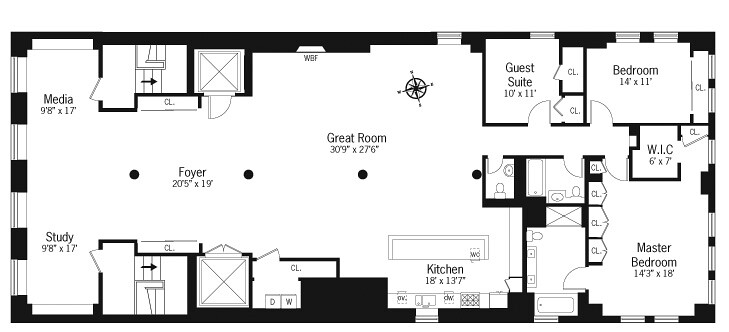Here is the cleaned-up and detailed caption for the blueprint image:

---

This blueprint illustrates the layout of a house, depicted as a large rectangular area with bold black lines denoting solid walls. White gaps represent either windows or doorways, with the doorways marked by angled openings.

Starting on the left-hand side, the blueprint features a media room and a study room, each measuring 9x8x17 feet. Both rooms have door openings that lead to flights of stairs, further leading into a foyer measuring 20.5x19 feet. The foyer contains two doors which may lead to elevators, indicated by square blocks with Xs.

Adjacent to the foyer is the great room, a spacious area measuring 39x27.6 feet, featuring a compass rose for orientation (northeast, south, and west).

Below and to the right of the great room, the blueprint reveals a kitchen measuring 18x13.7 feet. Exiting the kitchen to the right is an area that appears to contain two bathrooms. On the left side of this area, there is a guest suite measuring 10x11 feet and an adjacent bedroom measuring 14x11 feet.

To the right, the layout transitions into the master bedroom suite. This suite includes a master bedroom measuring 14.3x18 feet, a bathroom, and four small doors labeled "CL," indicating closets. Additionally, there is a walk-in closet measuring 6x7 feet.

---

This caption provides a clear, detailed description of the blueprint's layout, specifying dimensions and functions of each room while ensuring clarity for the reader.